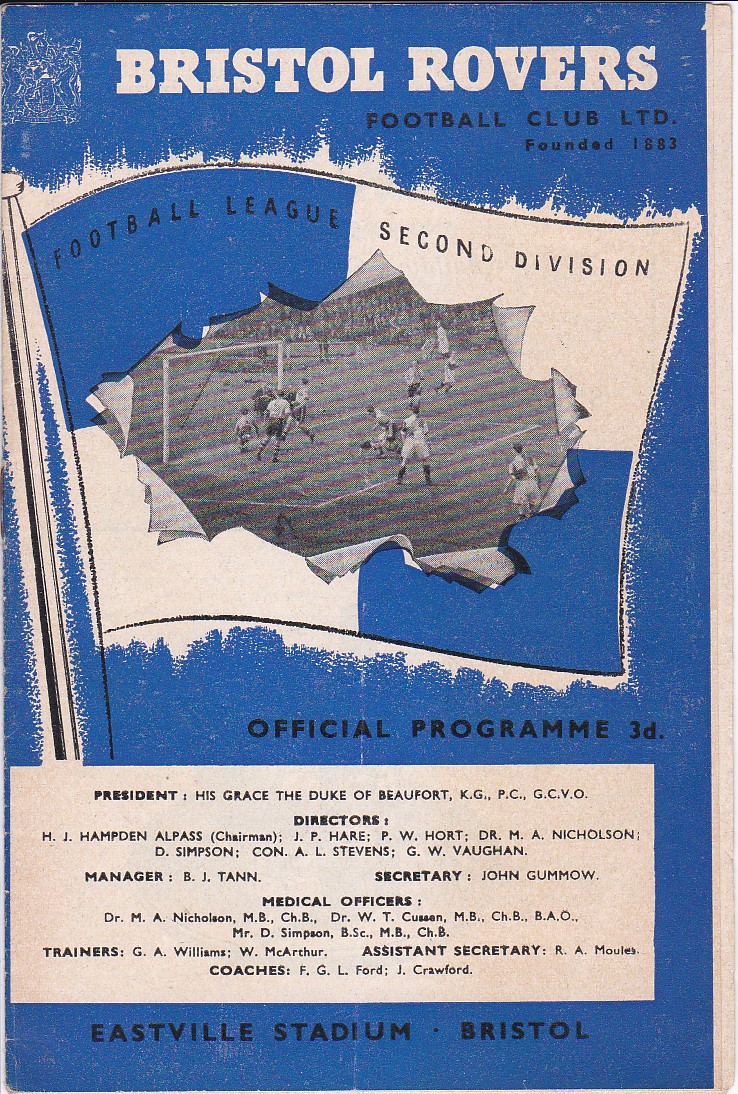This detailed description highlights an old, royal blue program for a soccer game featuring the Bristol Rovers Football Club. At the top, in large tan capital letters, it reads "BRISTOL ROVERS." Below, in smaller black letters, it states "Football Club Limited" and "Founded 1883." The central part features a tan flag, sectioned into four rectangles—upper left blue with "Football League" in black, upper right tan with "Second Division" in black, and the lower sections blank, with the center peeling back to reveal a black-and-white photo of a soccer match with several players on a field. Beneath the flag, in black capital letters, it says "OFFICIAL PROGRAM 3D." At the very bottom, "Eastville Stadium - Bristol" is printed over the blue background. Additionally, there's a tan rectangular section detailing club officials, including President His Grace the Duke of Beaufort KG, PC, GCVO, and lists of directors, managers, secretaries, medical officers, and coaches. Some names listed are H.J. Hamden-Allpast (Chairman), B.J. Tan (Manager), and Dr. M.A. Nicholson (Medical Officer). This artifact appears to be a meticulously detailed program from a past event held at Eastville Stadium.